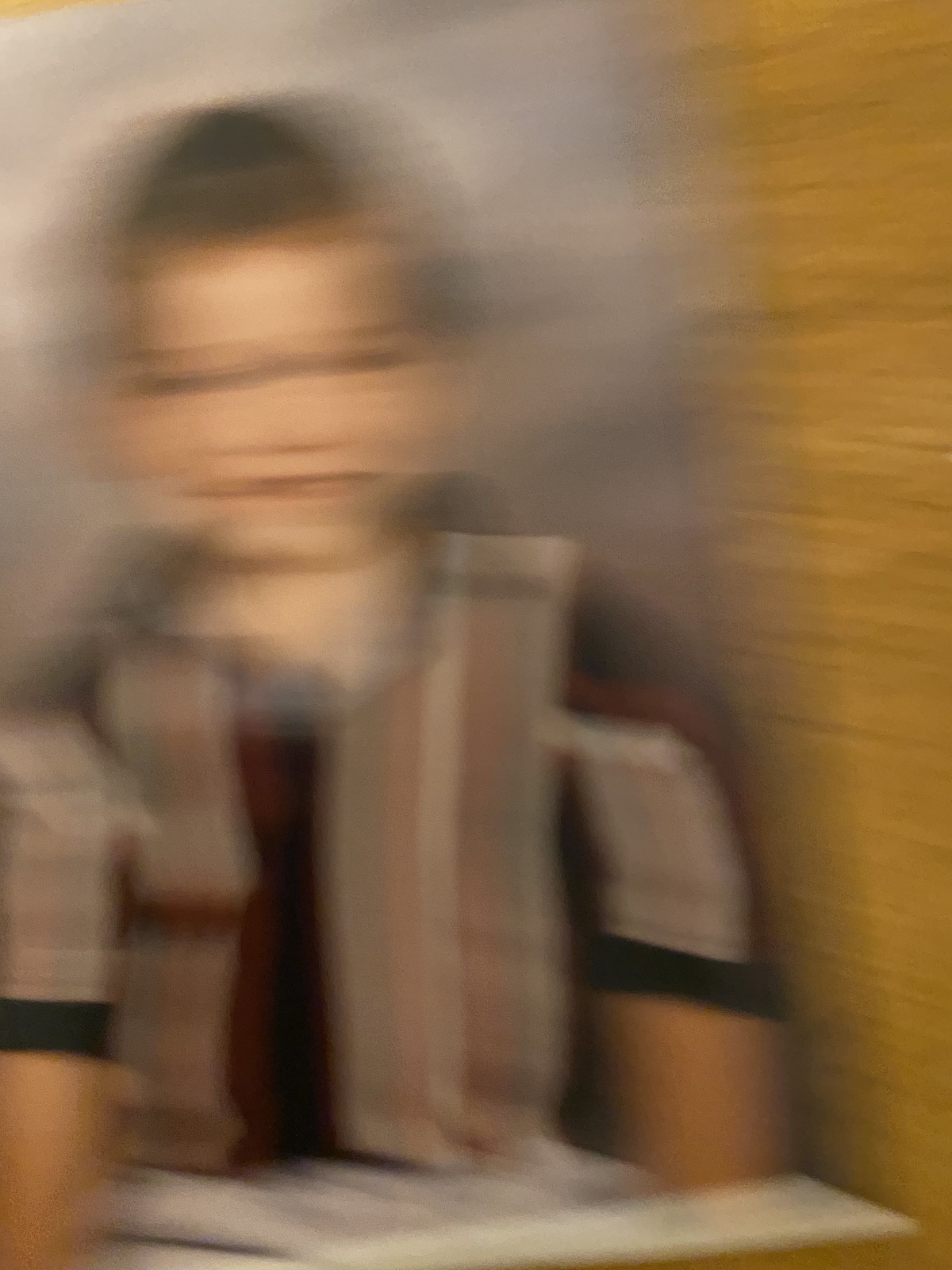This photograph features a young child with short brown hair and a bright smile. The child is wearing a vertically striped shirt with a vibrant mix of colors including white, pink, light blue, black, and maroon. To the right of the child is a brown-colored wall, providing a warm background contrast. In the foreground, partially obscuring the child, appears to be an open book, adding an element of curiosity and narration to the scene. The overall image is blurry, yet it captures the joyful essence of the moment.